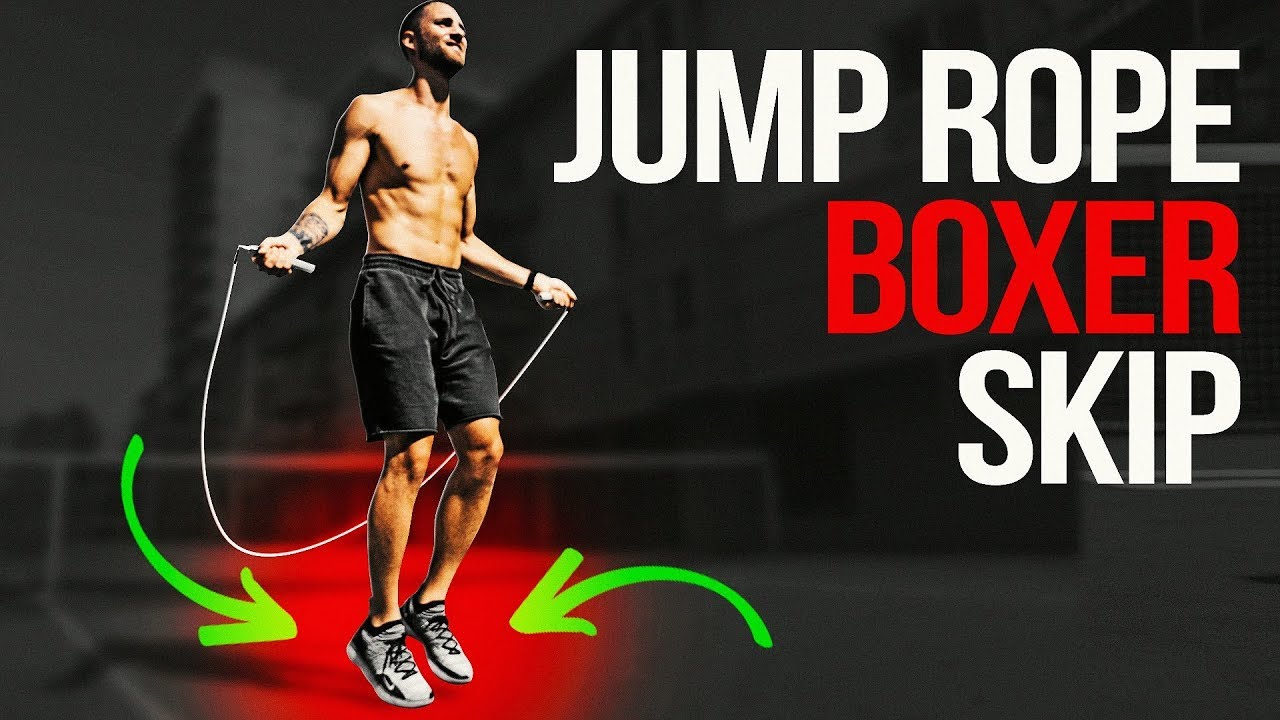The rectangular image features a color photograph of a Caucasian man jumping rope, set against a predominantly black background. The man, bare-chested and smiling, has short hair and is wearing black shorts and gray gym shoes. He holds a white jump rope, with green arrows digitally added to point at his feet in the mid-skip position. Notably, he has a tattoo on his inner right forearm and a watch on his left wrist. Above the man, in bold white print, the text reads "JUMP ROPE," followed by "BOXER" in red print, and then "SKIP" in all capital white letters beneath that. The writing is aligned along the right side of the image. A faint, almost building-like shadow appears behind the man, enhancing the impression that he is jumping outdoors.